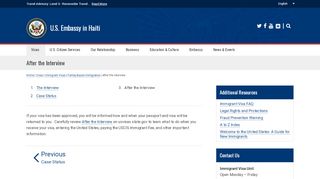A cluttered web browser screen is visible in this image, displaying multiple open tabs at the top, including the US Embassy in Haiti, Twitter, Facebook, and others. The webpage features a section labeled "Additional Resources," highlighted in blue, with five distinct lines of text beneath it. On the right side of the screen, there are five icons, presumed to be links or buttons. The top part of the page has a prominent blue bar, and the phrase "Contact Us" is present among the content. The overall webpage appears to be a resource or informational page from the US Embassy in Haiti.